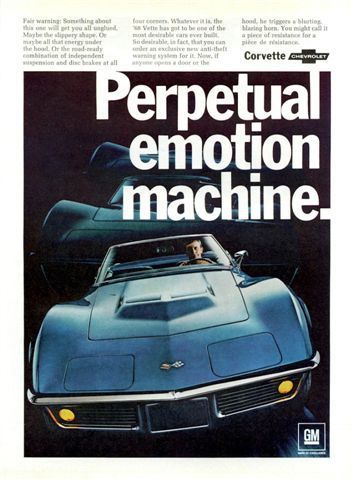This vintage magazine advertisement features a striking 1970s Corvette, set against a dramatic black background that evokes an impression of the car floating in outer space. The car, painted in a shimmering blue or bluish-gray hue, stands out vividly with its aerodynamic, sporty design. The distinctive front-on view reveals small yellow headlights and a chrome grille divided by a flat centerpiece, flanked by pronounced wheel flares. The Corvette, driven by an unseen man, also includes small side mirrors and a sleek, streamlined body. The headline, "Perpetual Emotion Machine," is emblazoned in large white letters at the top, with the GM logo visible in the lower right corner. Adding to the allure, ghosted, faded images of the Corvette linger in the background, emphasizing the car's timeless appeal and reinforcing its iconic status. Though the text at the top is too fine to read, it includes the Chevrolet logo and the word "Corvette," underscoring the car's brand heritage. The overall faded quality of the advertisement suggests it is from an era long past, enhancing its nostalgic and collectible value.